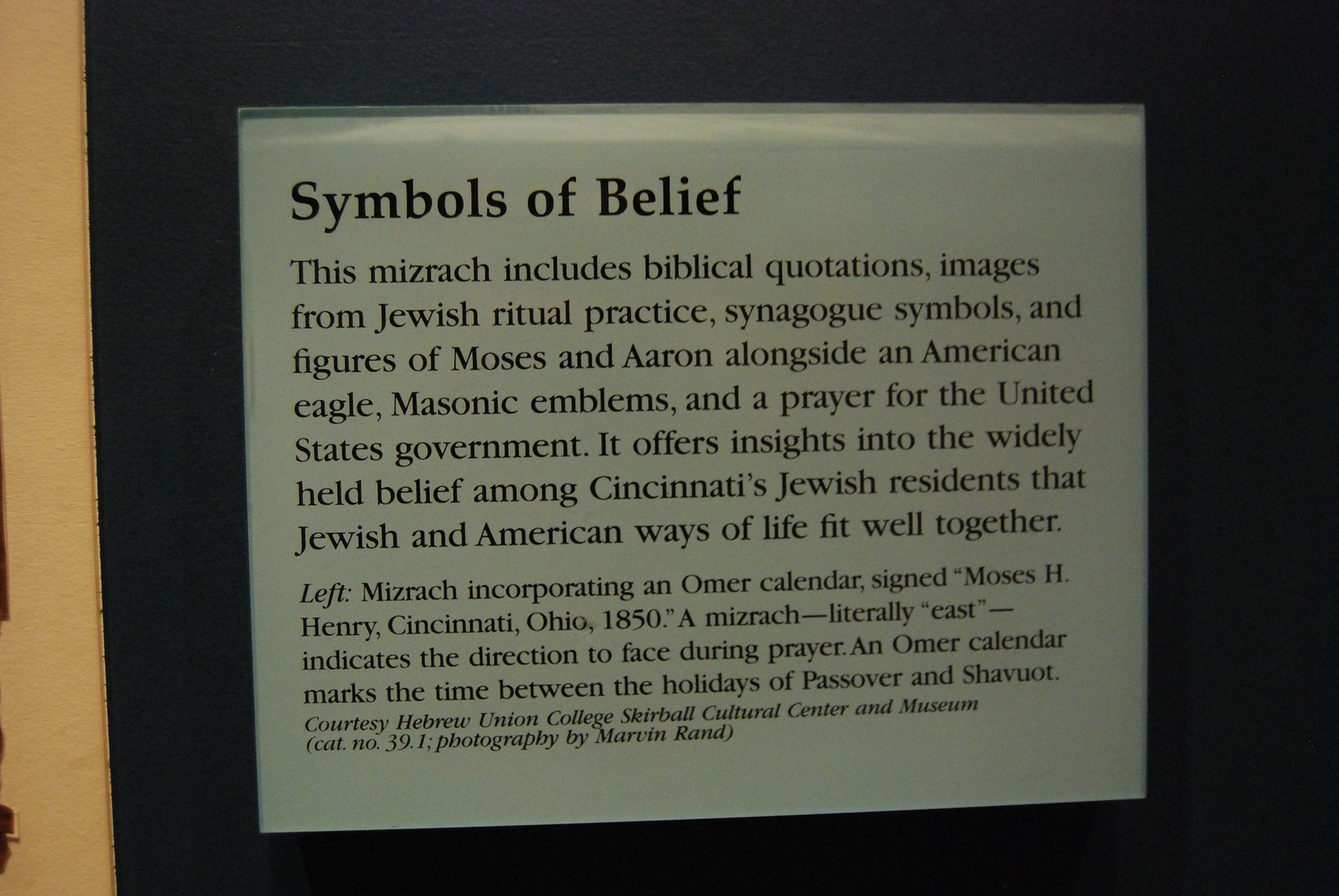The image depicts a laminated white sign hanging on a blue wall, possibly in a museum. Titled "Symbols of Belief," the sign provides detailed information about a mizrach, which includes biblical quotations, images from Jewish ritual practice, synagogue symbols, and figures of Moses and Aaron alongside an American eagle, Masonic emblems, and a prayer for the United States government. The mizrach offers insights into the belief held by Cincinnati's Jewish residents that Jewish and American ways of life are compatible. Additionally, the mizrach incorporates an Omer calendar signed by Moses H. Henry from Cincinnati, Ohio, dated 1850. The sign also explains that a mizrach, which literally means "east," indicates the direction to face during prayer, and that an Omer calendar marks the time between Passover and Shavuot. The information is courtesy of the Hebrew Union College, Skirball Cultural Center, and Museum, item number 39.1, with photography by Marvin Rand.